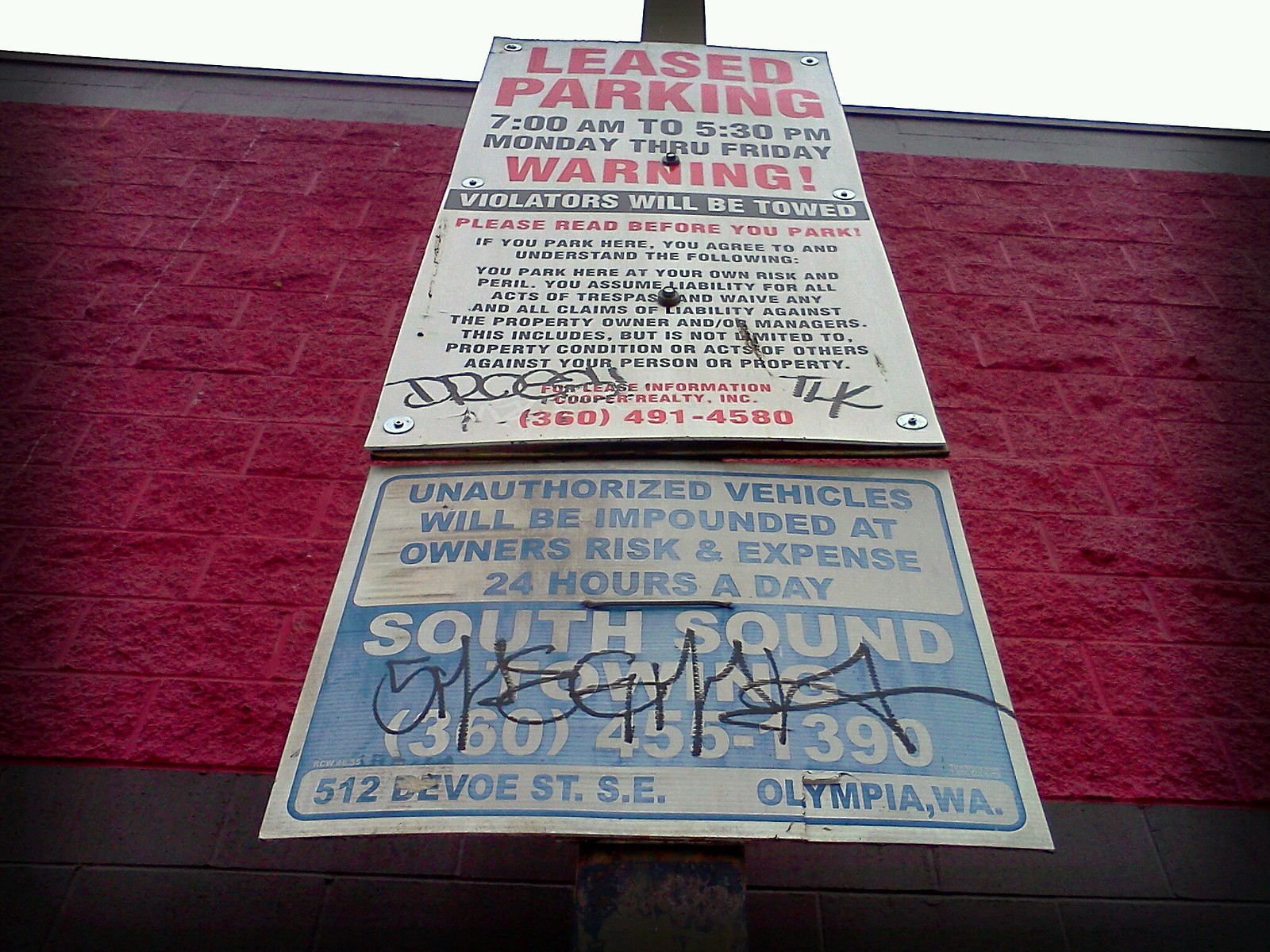This color photograph captures an upward view of two posted parking signs attached to a tall metal post. The signs are set against a backdrop of a cinder block building painted maroon, red, and black. The top sign is a long vertical white rectangle with various colored texts, primarily in red and black. The sign reads, “LEASED PARKING, 7AM TO 5:30PM, MONDAY THROUGH FRIDAY. WARNING! VIOLATORS WILL BE TOWED. PLEASE READ BEFORE YOU PARK.” Smaller black text below includes terms and conditions for parking, details of liability, and a contact number, 360-491-4580, associated with Cooper Realty, Inc. There's some graffiti on either side of the sign. The lower sign, which is white with blue text, states, “UNAUTHORIZED VEHICLES WILL BE IMPOUNDED AT OWNER'S RISK AND EXPENSE, 24 HOURS A DAY.” It provides the contact information for South Sound Towing, 360-455-1390, located at 512 DeVos Street SE, Olympia, WA, and is also marred with graffiti. The perspective angle that points the camera upward accentuates the height of the post and the layered textural details of the signs and the building.